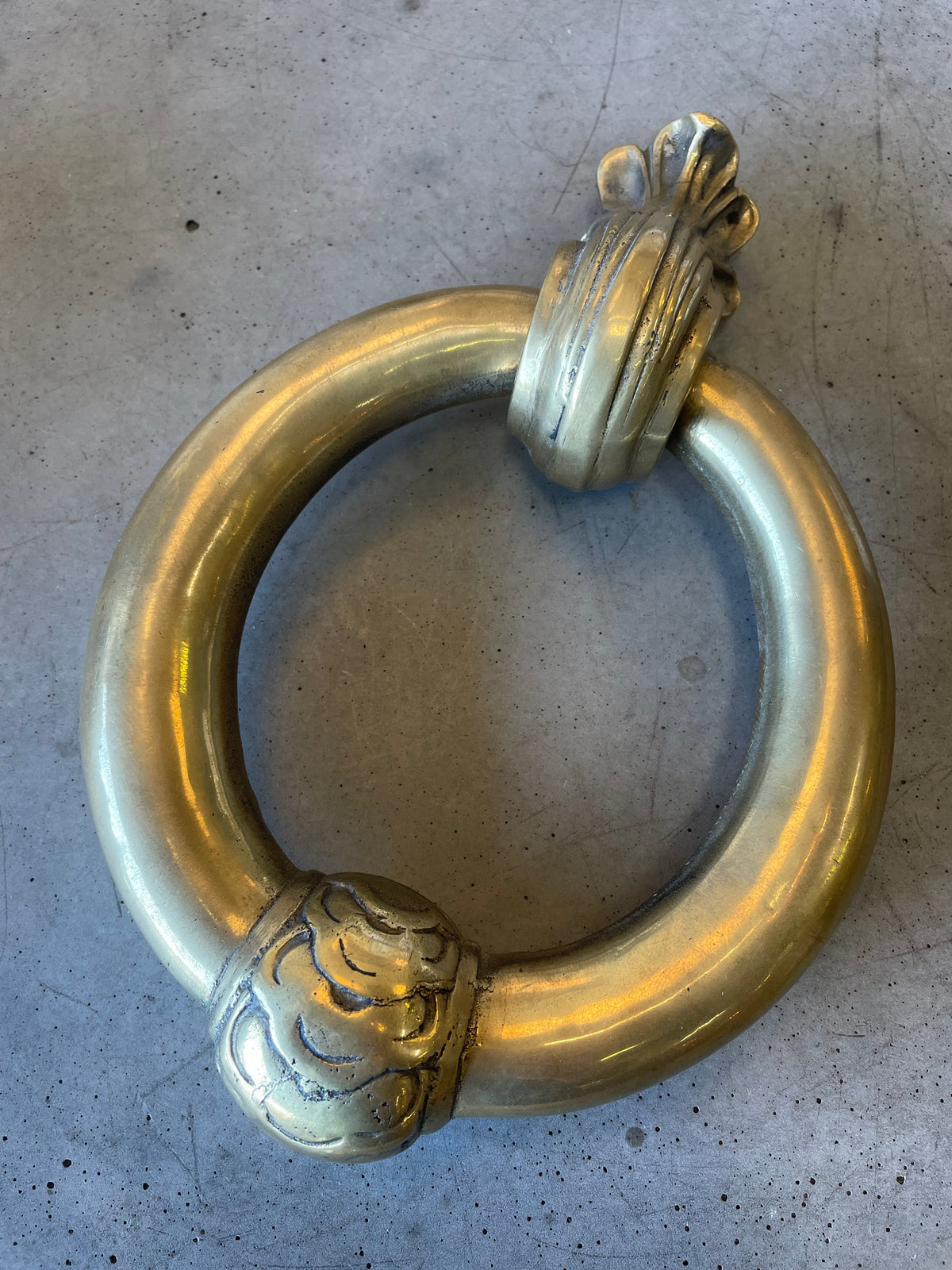The image depicts a close-up of a large, ornate gold ring resting on a mottled white and gray concrete surface speckled with black flecks. The ring appears exceptionally large, possibly intended for use as an ornament rather than a typical ring worn on a finger. 

Distinctive details adorn the ring: on the lower left side, there's a rounded section featuring three gold inlets with an intricate inlaid design that vaguely resembles a monkey face. On the upper right, a circular ornament with bands running across ends in two small protrusions resembling ears, with another larger, ear-like feature in the center, accented with gold and black inlays. The exquisite craftsmanship and detailed decorations suggest the ring may have a ceremonial or decorative purpose. The concrete background, with its unique texture, adds a stark contrast, making the gold ring’s intricate details stand out prominently.